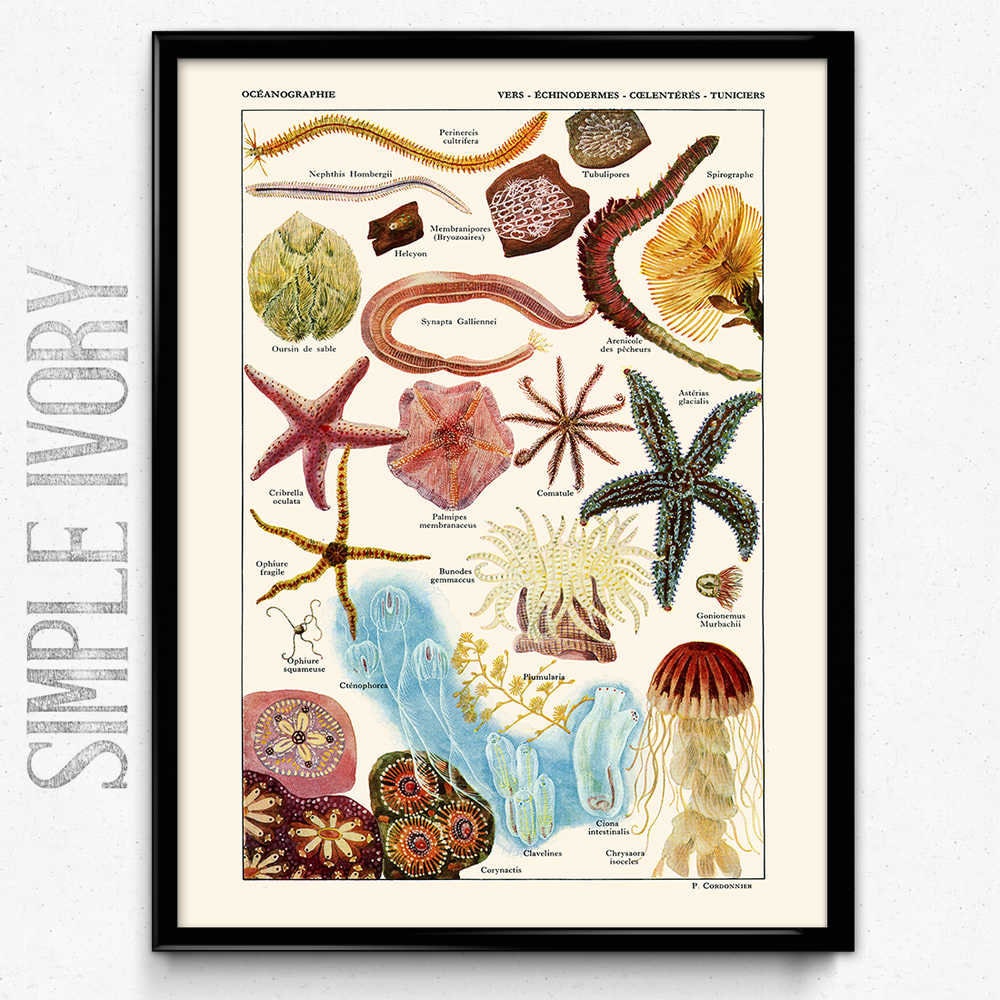The photograph displays a framed artwork against a predominantly white wall. The black picture frame encloses a detailed graphic with a white border inscribed with the word "Oshigraphy." Within this frame, intricate, scientifically labeled illustrations of various marine life forms are presented. Visible creatures include different species of starfish, eels, jellyfish, corals, bioluminescent organisms, and other sea dwellers. To the left of the main image, vertically oriented, bold, gray text reads "SIMPLE IVORY," slightly faded yet distinctly noticeable. The illustration of marine creatures showcases both traditional and unique species, all meticulously labeled with their scientific names.